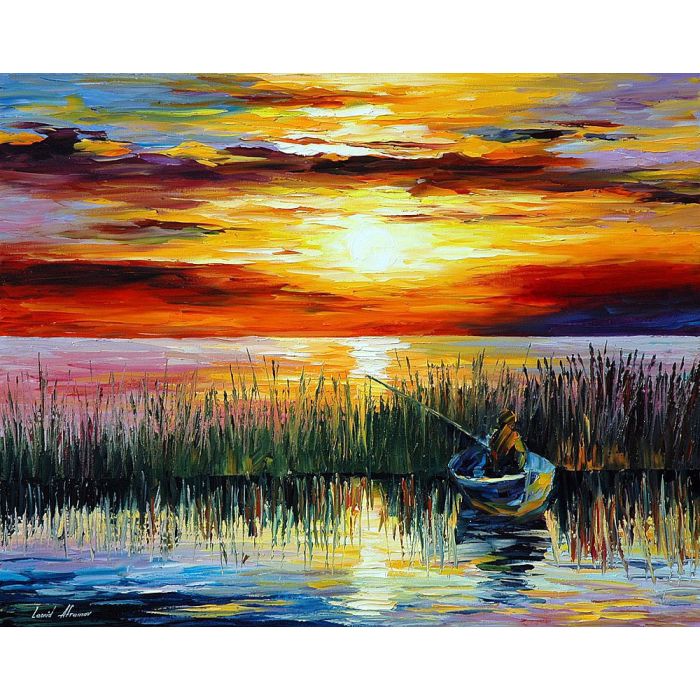In this vibrant and colorful oil painting, we see an artist's intricate depiction of a serene marsh area bordering a lake or larger body of water. The scene features a gentleman sitting in a small blue rowboat, surrounded by pussy willow reeds that vary in thickness and color—from thinner, greener stalks on the left to thicker, darker brown and black ones on the right. This reflective body of water is so smooth that it mirrors the boat, reeds, and the setting sun vividly. The gentleman, who may be either fishing or harvesting pussy willows, appears focused despite the absence of a clear fishing rod in one account, though one appears extending off the left side of the boat in another description.

The sky is a striking feature in this painting, showcasing a stunning palette as the sun sets just above the horizon. The sun itself shines a bright white in the center, with golden hues radiating outward. Ribbons of clouds stretch across the sky, illuminated in shades of orange, red, and purple, with a prominent dark line of cloud contrasting against the bright orange and yellow gradient near the horizon. The sunlight casts a warm glow onto the water, enhancing the tranquility and beauty of the marsh. In the distance, possibly on the far side of the larger body of water, there appears to be a dark shoreline, subtly highlighted in purples and blues, adding depth to the composition and emphasizing the peaceful isolation of the man in his boat.